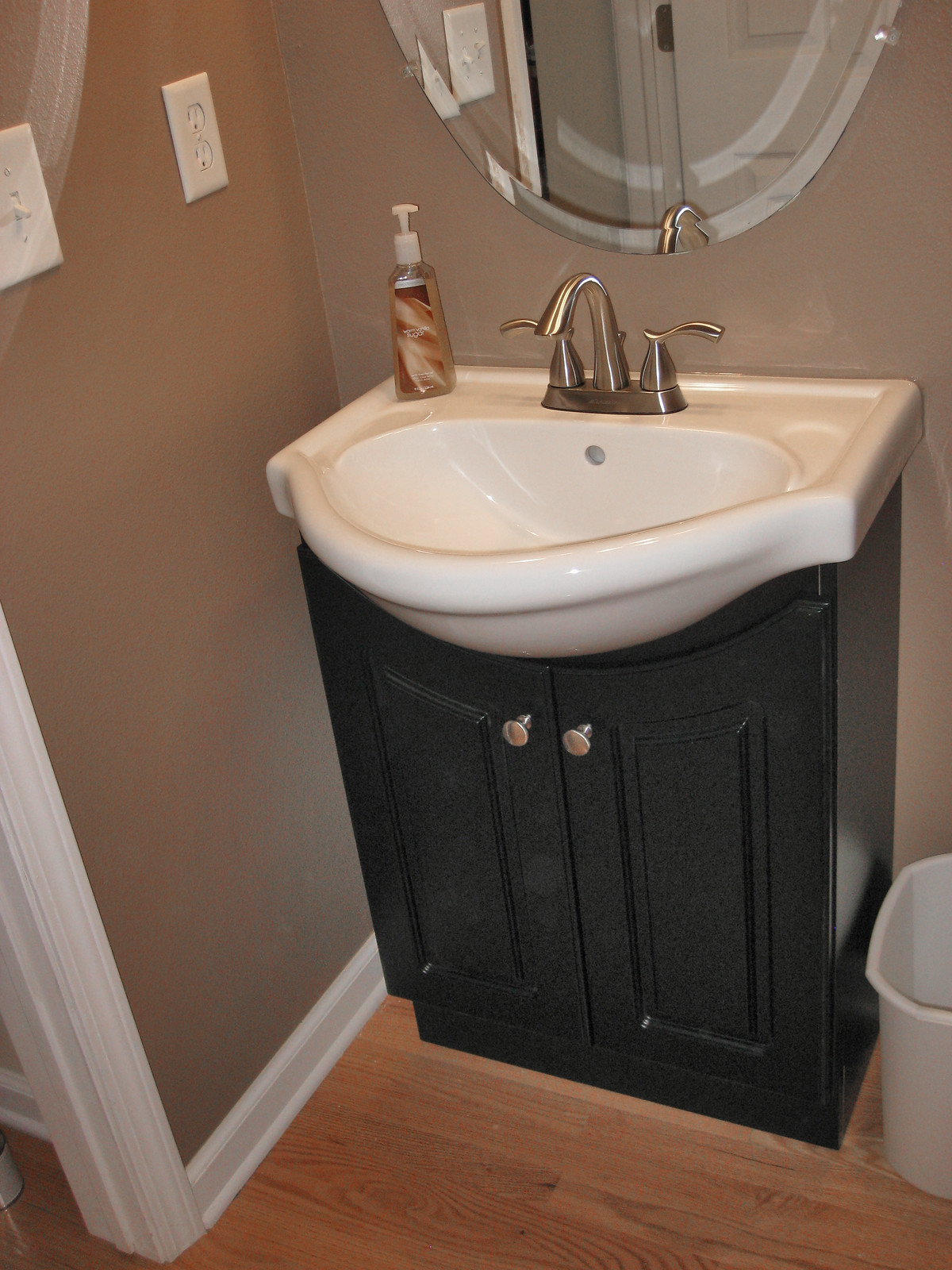A vertical photograph captures a tastefully designed bathroom corner, emphasizing the room's sophisticated elements. The floor features light wood slats, showcasing noticeable grain details that add a natural touch to the space. The walls are painted in a shade that can be described as either a very dark beige or a light brown, contributing to the room's warm ambiance.

A significant portion of the scene highlights a doorway with white trim, likely leading to another section of the bathroom. Adjacent to the doorway, there is a crisp white light switch and a double plug power outlet.

The focal point of the image is a sleek black vanity, equipped with a white sink and a nickel-colored faucet. The vanity's cabinet doors feature two handles, adding a subtle contrast to the overall color scheme. Atop the vanity rests a bottle of hand soap, ready for use. Above this setup, a round mirror is prominently displayed, offering both function and a touch of elegance.

To the right of the vanity, limited counter space is available for placing small items, ensuring the area remains uncluttered. On the floor, a white trash bin completes the scene, maintaining the bathroom's clean and orderly appearance.